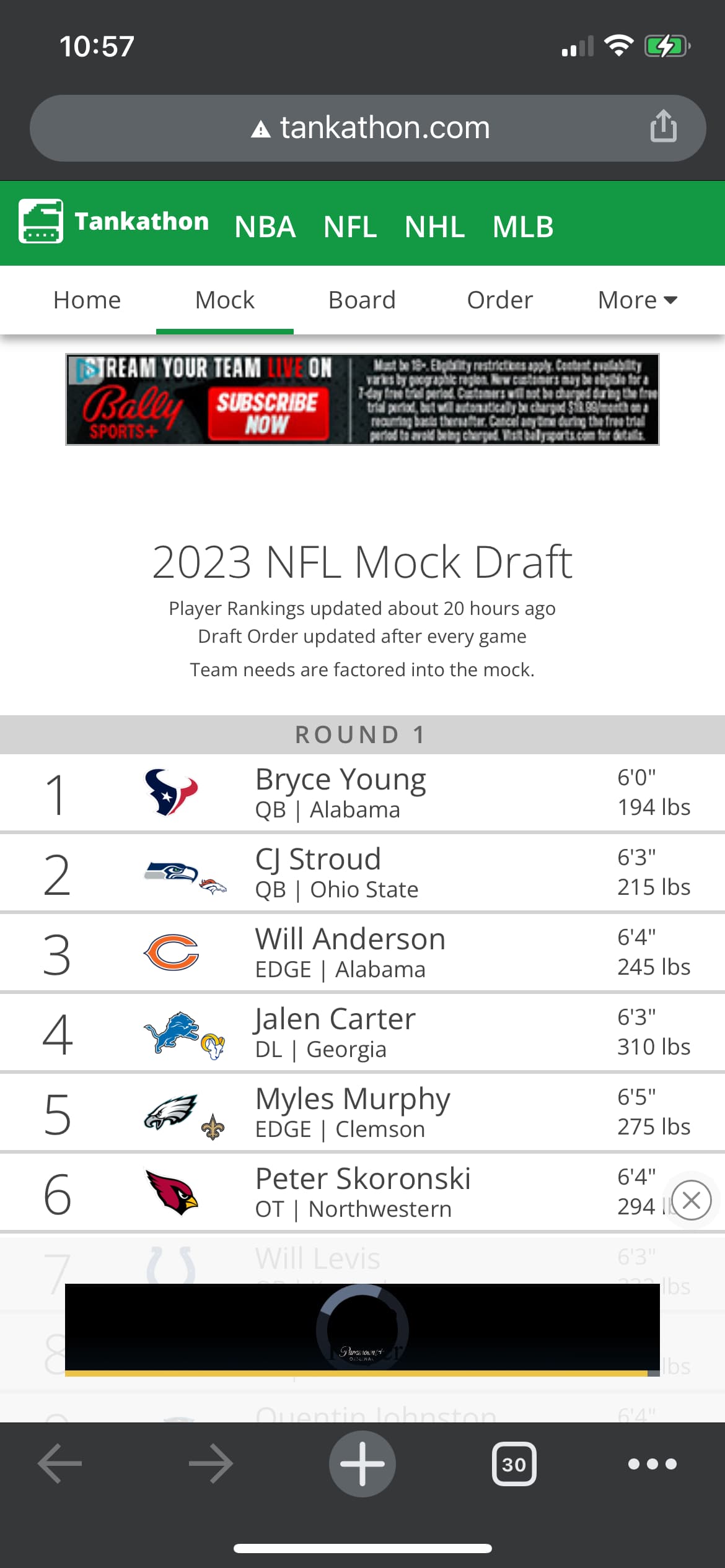The mobile screen is viewed in portrait mode and shows the website tankathon.com in the top left corner. The top status bar indicates the time as 10:57 AM on the right side. There are two bars of cell signal alongside the Wi-Fi signal, and a full green battery icon with a lightning bolt in the middle signifying it's charging.

The website's URL bar is long and circular, featuring a green strip with the word "tankathon" and a green tank logo on a white square background to the left. Adjacent to these are the labels for different sports leagues: "NBA," "NFL," "NHL," and "MLB." To the right, a white menu bar lists "Home" and "Mock" in black lettering, with a green line highlighting "Mock." Additional menu options include "Board," "Order," and "More" with a dropdown arrow.

Below the menu is a dark gray advertisement for Bally Sports Plus, featuring a red logo and white text with smaller white writing towards the right.

The main content area displays the title "2023 NFL Mock Draft Player Rankings," updated about 20 hours ago. It mentions that the draft order is updated after every game and team needs are factored into the mock. The section titled "ROUND 1" is highlighted with spaced letters and a light gray rectangular border. The draft order lists:
1. Bryce Young
2. CJ Stroud
3. Will Anderson
4. Jalen Carter
5. Myles Murphy
6. Peter Skowronski.